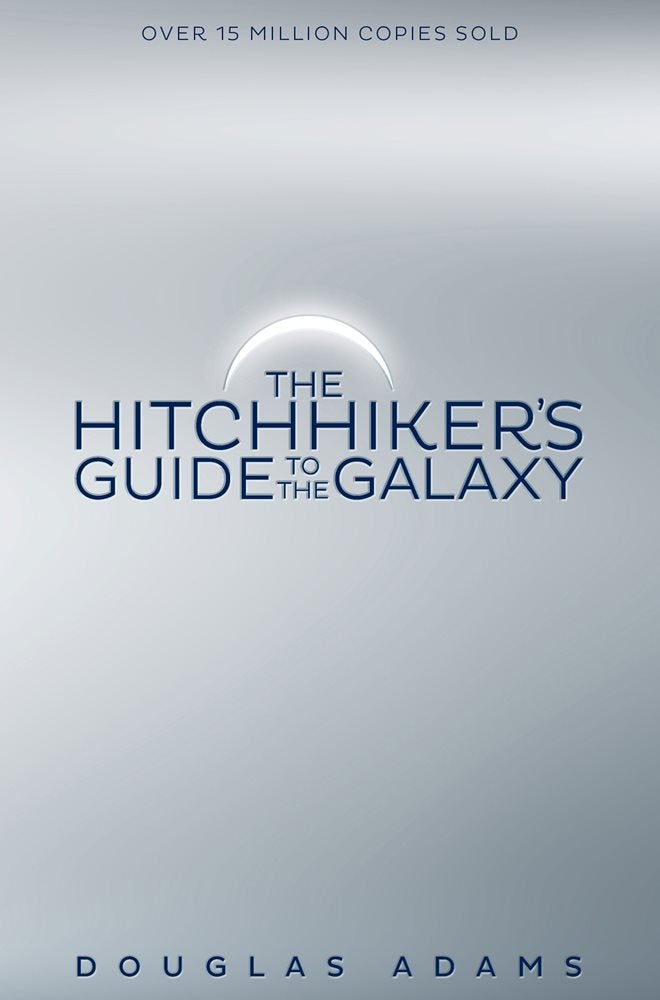The book cover of "The Hitchhiker's Guide to the Galaxy" by Douglas Adams features a predominantly grayish-blue backdrop with shades resembling starlight, blending both blue and white hues. At the very top, the cover prominently announces, "Over 15 million copies sold" in dark blue font. Centrally located is the title, "The Hitchhiker's Guide to the Galaxy," also in dark blue. Over the word "THE" in the title is an arcing crescent moon, adding a whimsical touch. At the bottom of the cover, the author's name, Douglas Adams, is displayed in the same dark blue font as the other text. The overall design transitions from lighter shades at the top to slightly darker tones at the bottom, creating an elegant and visually appealing book cover.